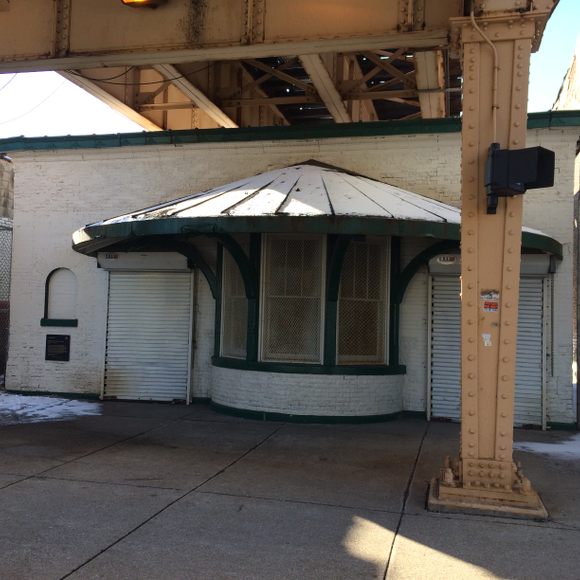This photograph depicts a white brick building situated beneath a yellow, riveted railway bridge, evocative of the industrial platforms found in cities like Chicago or New York. The building prominently features a trio of large, curved windows that project outward, sheltered by a green awning dusted with snow. Flanking these bay windows are two tall, narrow white metal garage doors. Adjacent to the left garage door, there's a small, arched window with a black plaque positioned below it. The edifice is capped with a green roof, and large concrete slabs pave the area in front. A robust pillar supporting the yellow railway bridge is visible on the right side of the image, adding to the structure's urban, industrial character.